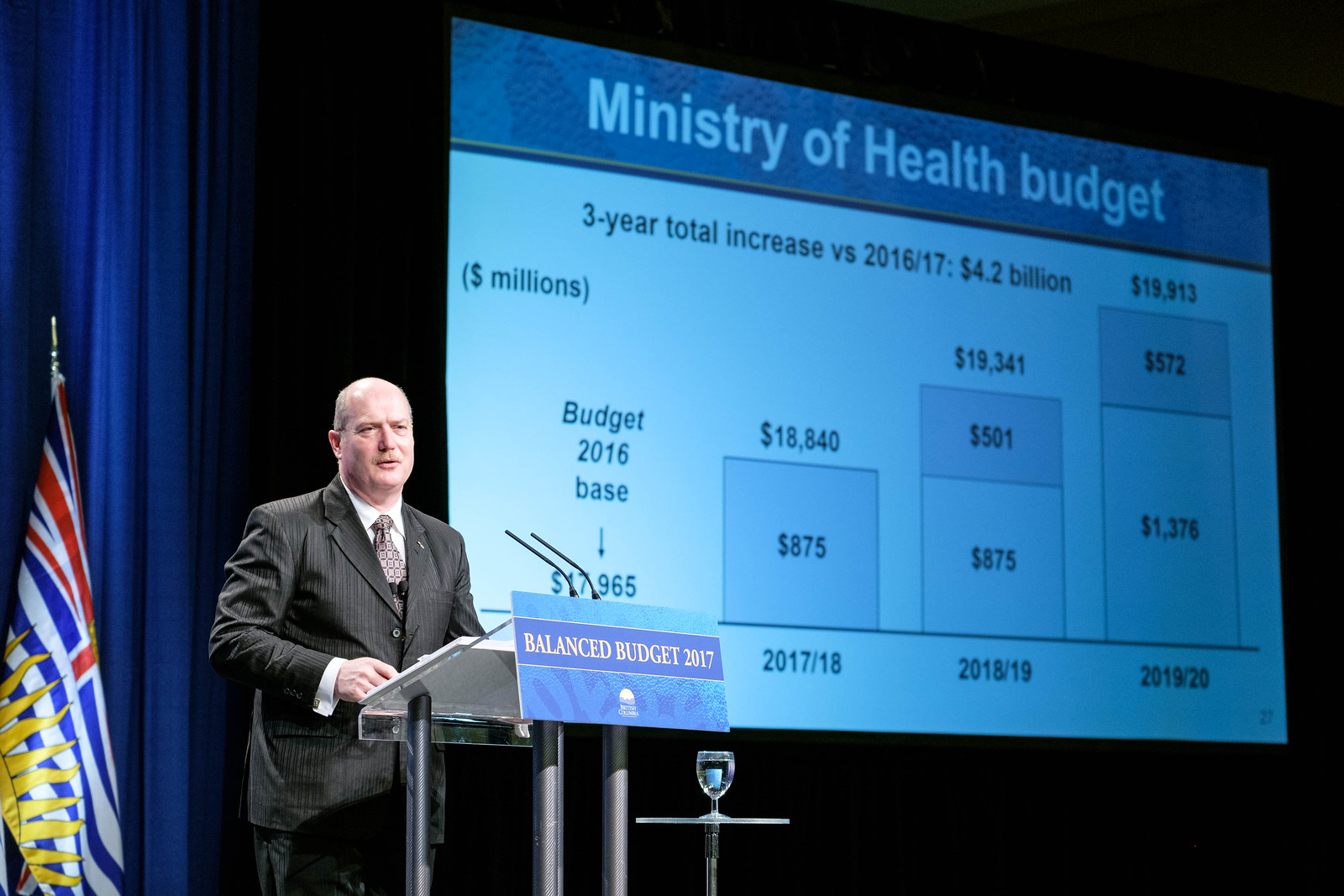A balding middle-aged man in a striped blue suit and tie stands at a gray, acrylic podium during a speech. Clipped to his lapel is a microphone. In front of the podium is a sign that reads "Balanced Budget 2017, British Columbia," with a British Columbia logo at the bottom. Behind him, a large projection screen displays a presentation titled "Ministry of Health Budget." The screen shows a detailed bar graph illustrating a three-year total increase of $4.2 billion compared to the 2016-17 base, with figures rising from $17,965 in 2016 to $19,913 by 2019-20. The backdrop is predominantly black with blue curtains, and to the right, a flag featuring red, white, blue colors, and a yellow sun is visible. In the foreground, a small table holds a glass of water.